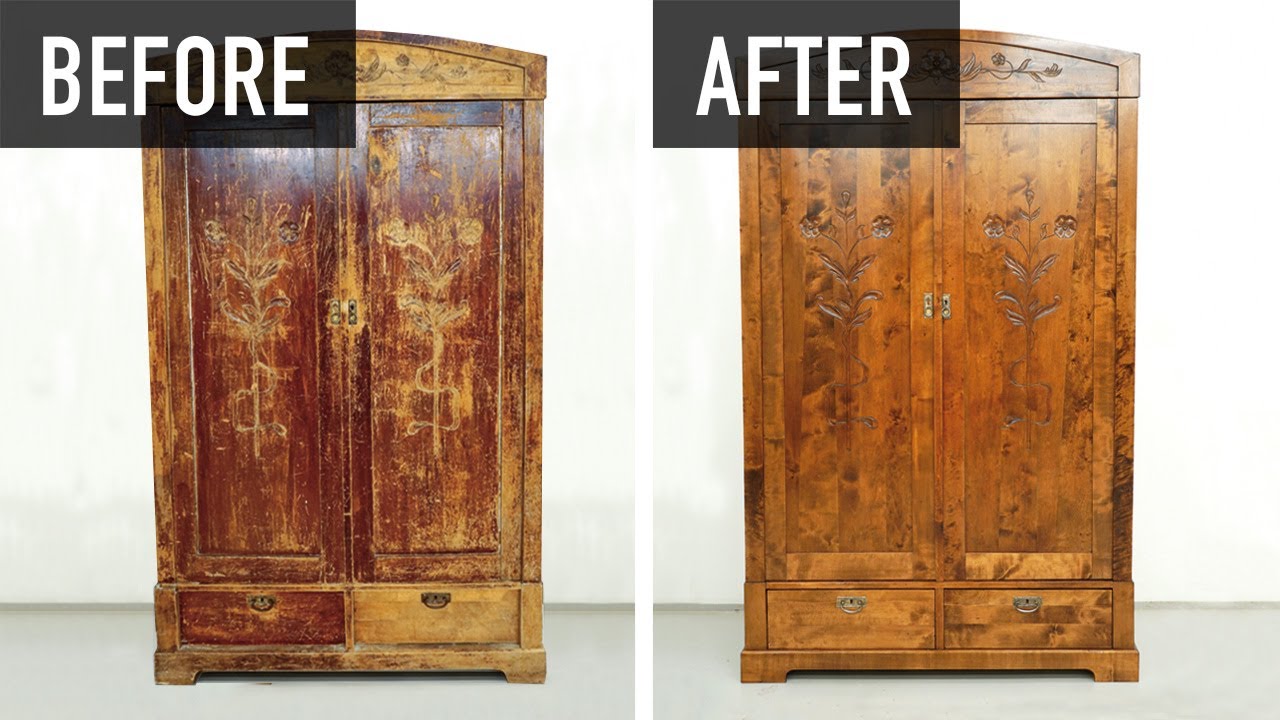The image is an advertisement for furniture repair, showcasing a dramatic restoration of a tall, wooden dresser. Divided by a white line, the left side features the heavily worn dresser labeled "BEFORE" in a big black box with bold white letters, while the right side displays the pristine, restored dresser labeled "AFTER" in a similar black box. The "BEFORE" picture reveals extensive scratches, uneven coloration with light and dark patches, dry and aged wood, and missing paint on the top. The dresser, positioned against a white wall on a gray floor, has two drawers at the bottom and double doors with decorations. In stark contrast, the "AFTER" image shows the dresser beautifully restored to a uniform color, shiny, vibrant, and free of any damage or distortion, highlighting the remarkable transformation.